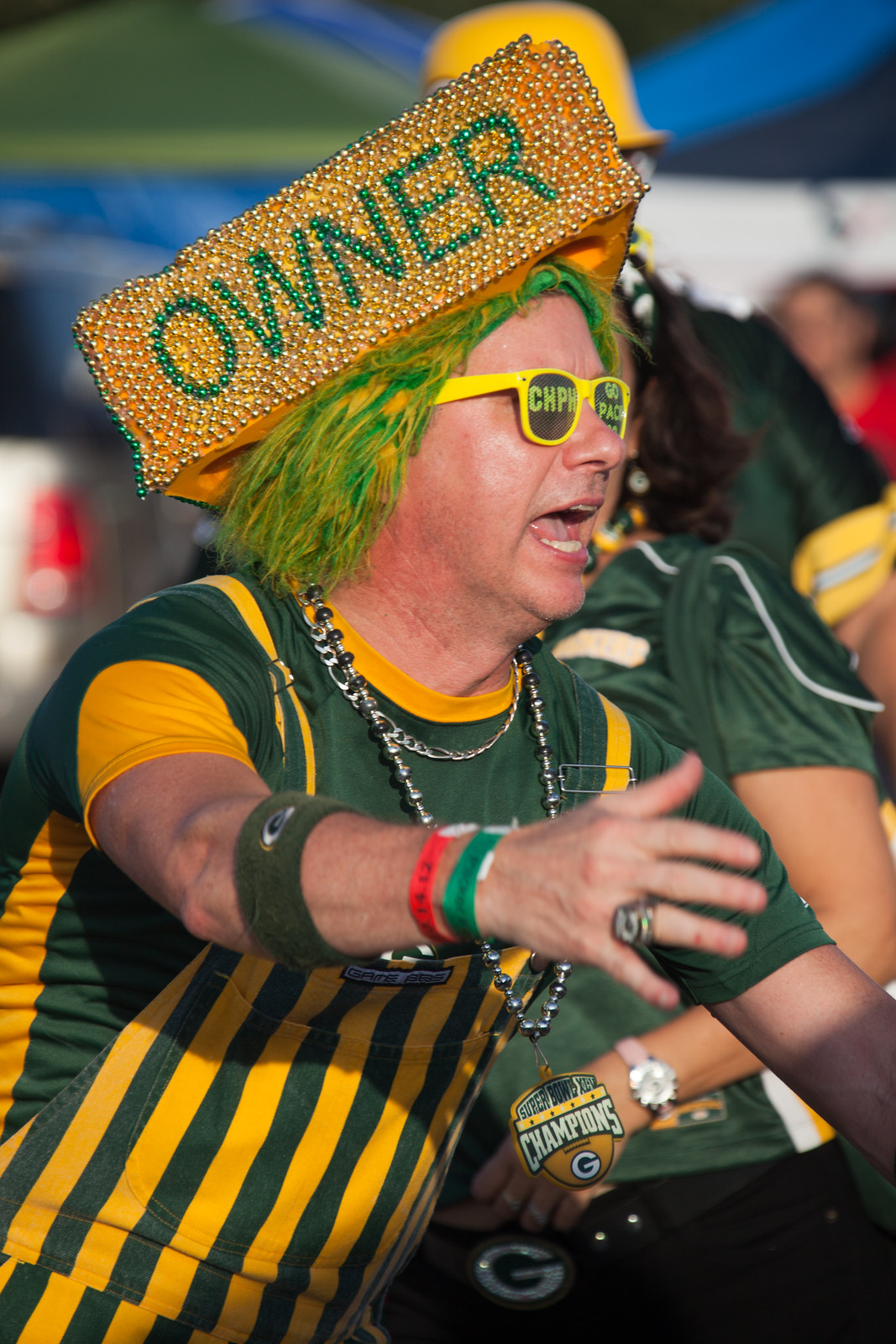The image features an exuberant Green Bay Packers fan immersed in the game-day spirit. Sporting a tall, bejeweled cheese wedge hat with the word "Owner" prominently displayed in sparkling beads, the fan's vibrant outfit captures attention. A green and yellow shoulder-length wig flows beneath the hat, matching the team's colors perfectly. The fan's bright yellow mirrored sunglasses add an energetic flair to his animated expression, as he appears to be either cheering or yelling passionately. 

His attire includes a green T-shirt layered under green and yellow vertically striped bib overalls, epitomizing team pride. Accessorized with a red and green wristband, a Packers armband, and a robust necklace featuring a silver chain with a pendant declaring "Super Bowl Champions" adorned with the Packers' "G" logo, the fan is decked out from head to toe. 

The background hints at the bustling stadium atmosphere, though it remains blurred, showcasing more fans, including one in a yellow hard hat and another possibly in a red T-shirt. Overall, the image paints a lively picture of unbridled enthusiasm and dedication to the Green Bay Packers.